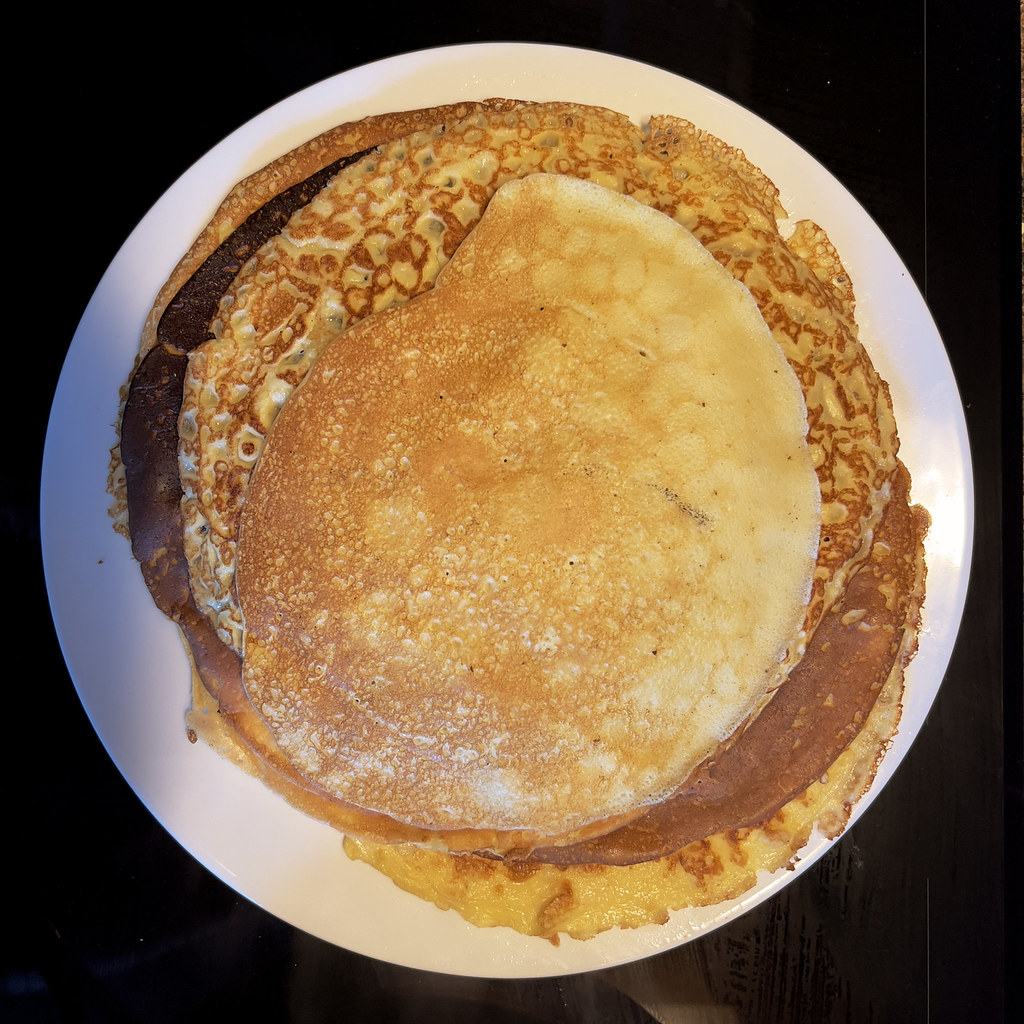A bird's-eye view captures a stack of golden brown pancakes arranged on a round white plate, situated on a dark brown wooden table. The plate, which is set against a predominantly dark background that shifts from black in the top left corner to brown in the lower right, holds between four to seven pancakes, their exact number indistinguishable from the aerial perspective. The pancakes vary in size and consistency; some exhibit a light golden color with whitish edges, whereas others are darker, with the one second from the bottom appearing slightly burnt. The pancake on the top is notably smaller and has an uneven shape with a smooth, circular edge on one side, contrasting with a misshapen edge on the other. The detailed textures and colors of the pancakes, ranging from light tan to deep brown, are accentuated by the focused, close-up shot.